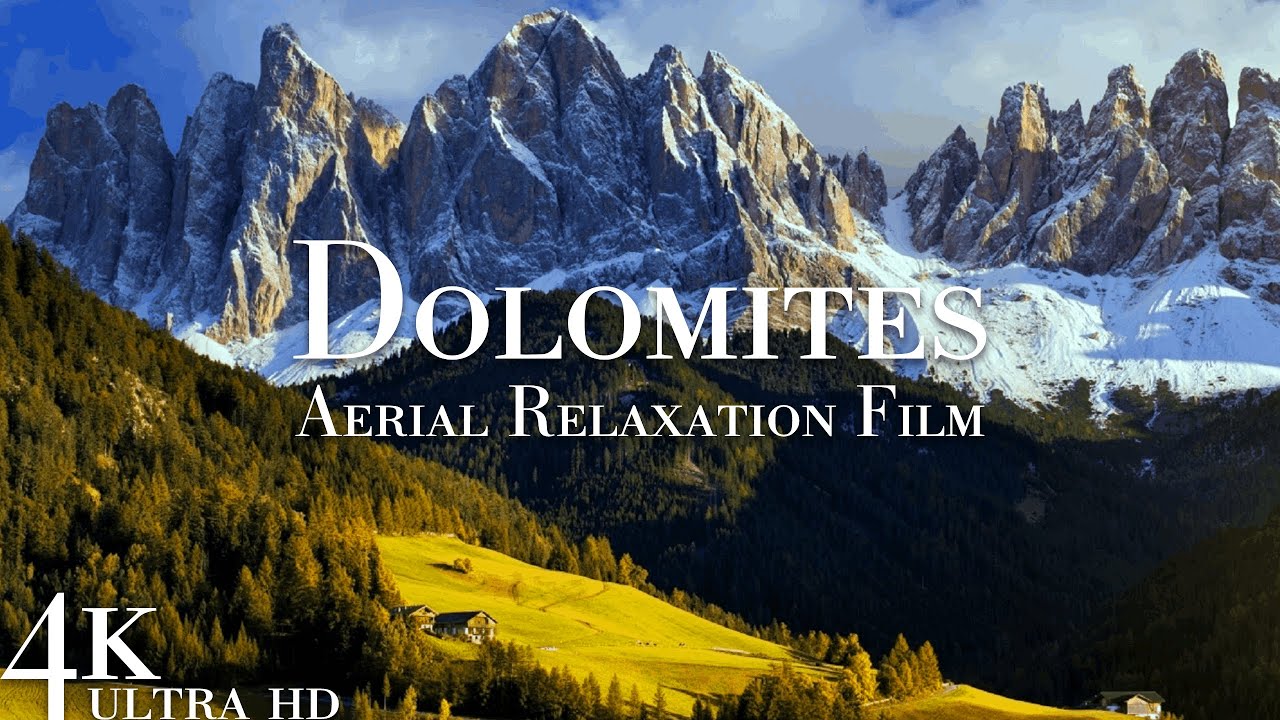The image is a stunning advertisement for a movie titled "Dolomites Aerial Relaxation Film," prominently displayed in large white text at the center of the scene. The breathtaking photograph showcases the majestic Dolomites mountain range, characterized by its towering, angular peaks dusted with snow, which glisten under a bright blue sky adorned with beautiful clouds. The rugged, barren peaks transition seamlessly into lower mountains covered in lush green pine forests. In the foreground, the landscape softens into a vast valley of verdant pastures and meadows, speckled with fields of green and yellow grasses. Nestled within this picturesque valley are two small houses—one to the bottom left and another to the bottom right—offering an idyllic and serene living experience with spectacular views. The bottom left corner of the image additionally features the label "4K Ultra HD," indicating the high-definition quality of the film, enhancing the immersive experience of this natural wonder.